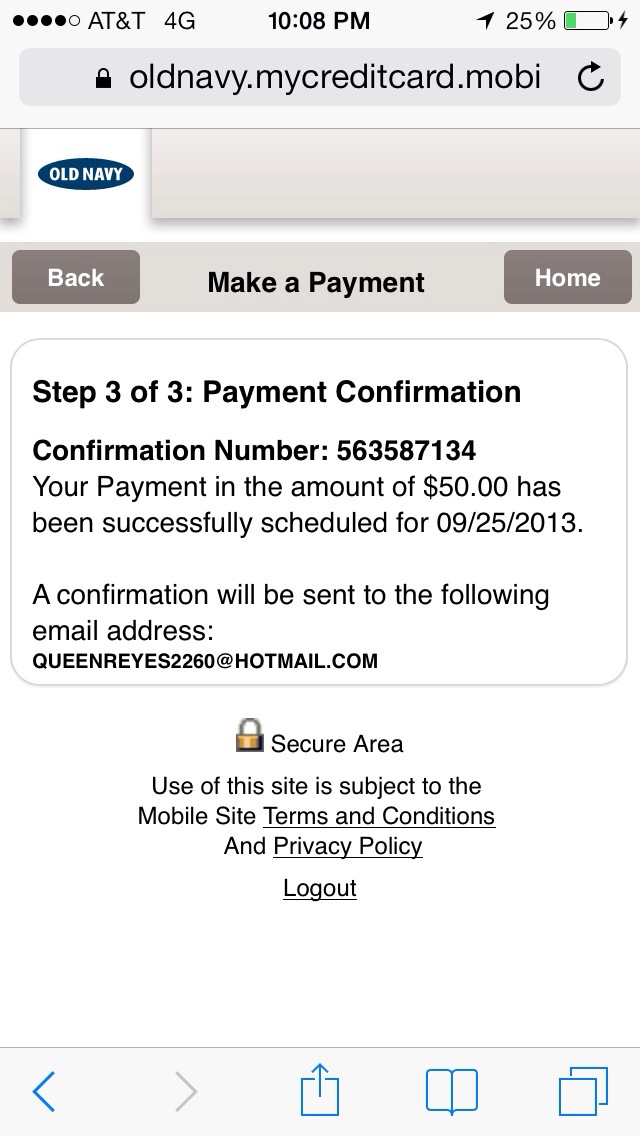This image captures a screenshot from a smartphone displaying a mobile payment confirmation on the Old Navy credit card website, oldnavy.mycreditcard.mobi. At the very top of the screen, a gray banner features a padlock icon next to the website address, and an arrow symbol indicating a loading or refresh action. The device shows it's connected to AT&T 4G network at 10:08 p.m. with a 25% battery level and 4 out of 5 signal bars.

Beneath this, another gray banner displays the recognizable Old Navy logo—a blue oval with white text. This banner is flanked by a dark gray "Back" button on the left and a white "Home" button on the right, all situated below a light gray section that reads "Make a Payment" in black text.

The bulk of the screen is white, containing detailed payment information. It states "Step 3 of 3, Payment Confirmation." Below, a confirmation number "563587134" is provided, indicating that a payment of $50 has been successfully scheduled for September 25, 2013. The confirmation will be sent to the email address cleanreyes2260@hotmail.com. Additional sections indicate that the user is in a secure area, marked by a gold lock icon, and there are links to the mobile site's terms and conditions, privacy policy, and a logout option at the bottom.

This detailed visual account provides a complete view of the payment confirmation process on the Old Navy credit card mobile site, with clear navigational elements and user-specific transaction details.